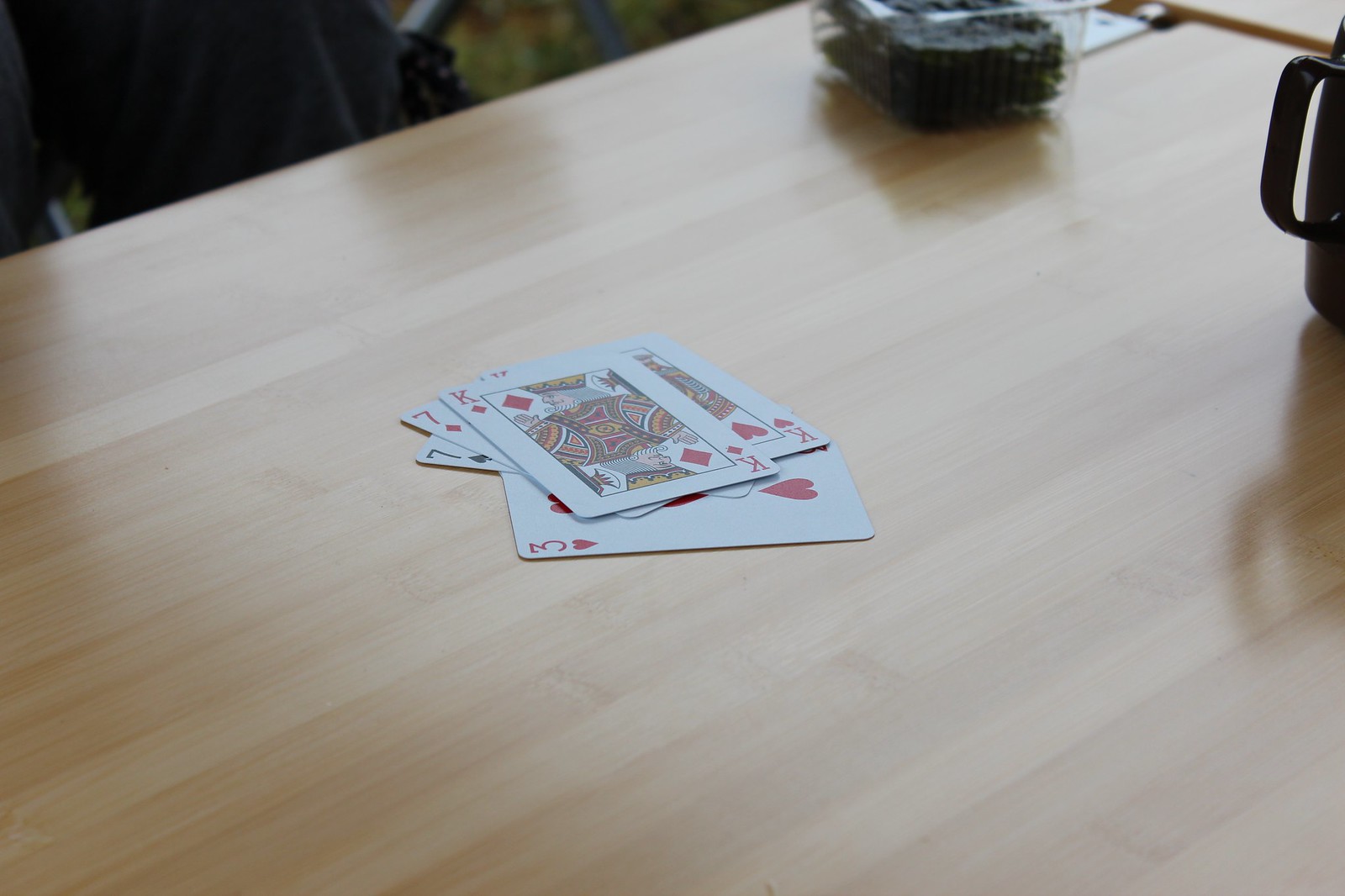In the center of the image, there is a small stack of five plain playing cards fanned out in a slight swirl pattern on a light brown rectangular table. The table's surface features slanted lines running across it. The playing cards themselves sport a white background and depict two kings, two sevens, and a three. To the right of the card stack, there is a tall black coffee mug or possibly a pot, with the handle and rim clearly visible. In the upper left corner of the image, a plastic bowl or container holds thin strips of dark seaweed, predominantly black with hints of dark green along the edges. To the far left, a person is partially visible, seated and wearing dark gray pants, though specific details of the individual are unclear.